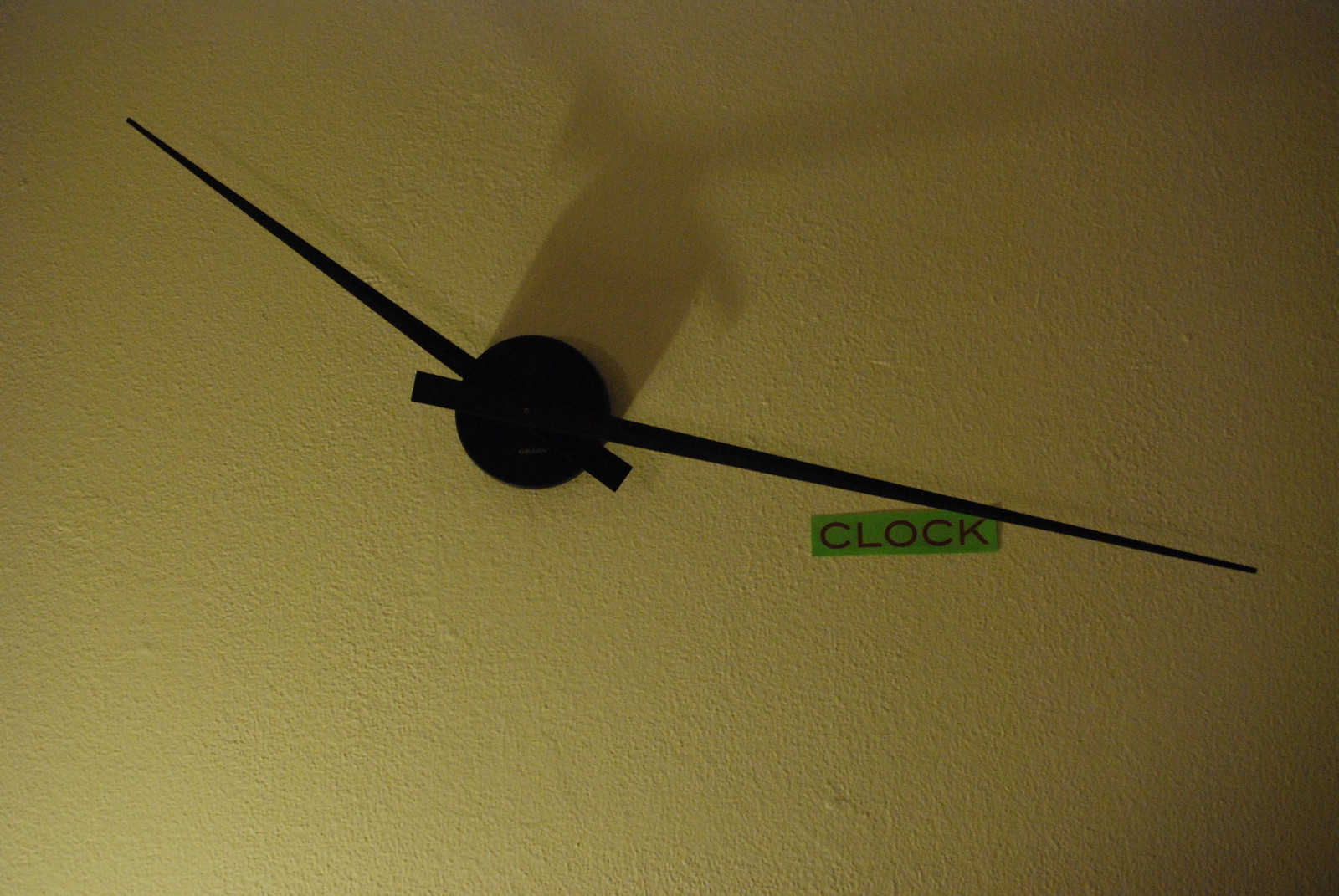This indoor photograph captures a minimalist clock attached to a pale yellow wall. The clock consists solely of a small, round base with two hands—the minute and the hour hand—without any numbers or background. Light from a lamp in the lower left corner casts pronounced shadows upwards and to the right, adding depth to the otherwise mysterious and dark image. A small green label with the word "CLOCK" written in red is taped nearby, suggesting the purpose of the mechanism. The overall simplicity and lack of traditional clock elements give the image a quirky, almost humorous vibe.